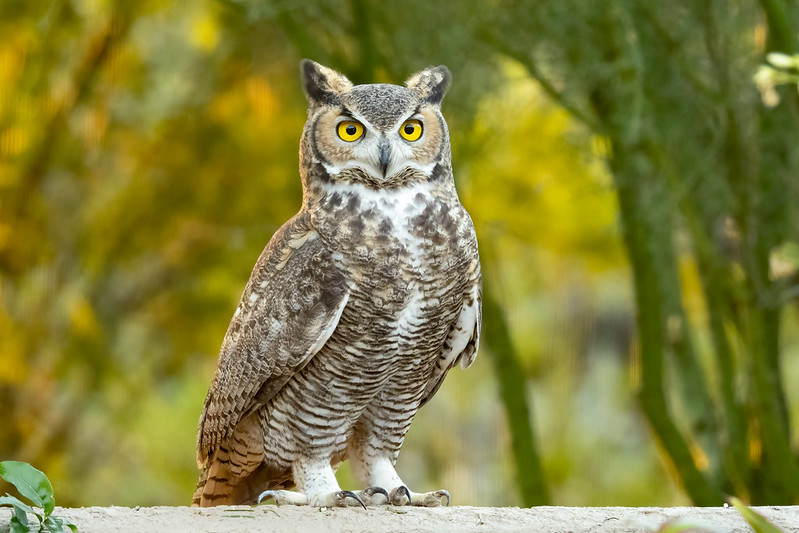This detailed photo captures an owl perched on a light gray log, set against a strongly blurred background that emphasizes the owl's intricate features. The backdrop displays tree branches and lush greenery, adding a vibrant, natural hue to the image. The owl's feet are bright white, adorned with long, sharp talons curved downward, ready to catch prey. Its breast is decorated with brown and white striped feathers, while its wings showcase a predominantly brown color with scattered white spots. The tail feathers are tan with brown striping, contributing to a textured appearance. The owl's head is striking, featuring vibrant yellow eyes surrounded by light brown feathers, a dark gray area near the beak, and ears with a mix of black and tan. Overall, the primary color of the owl is brown, accented by white and some black, creating a harmonious yet detailed plumage.